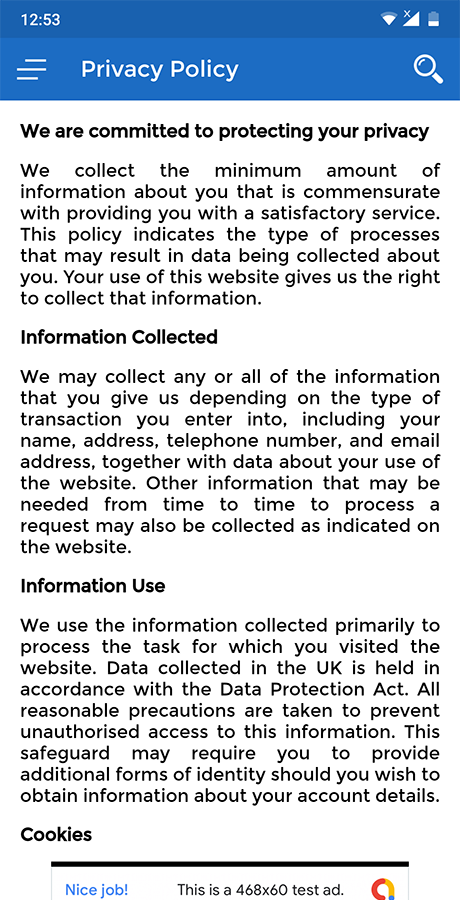A detailed description of the image would be:

---

The image shows a screenshot of a company's privacy policy as seen on a mobile device. At the very top of the screen, there is a blue border displaying the current time, 12:53 PM. To the right of the time, the status icons indicate a strong Wi-Fi connection, full signal for mobile data, and a battery level at one-third capacity.

Directly below the blue border, the interface includes a white search magnifying glass icon on the right and a three-horizontal line menu icon, indicating additional options. Adjacent to these icons, the heading "Privacy Policy" is prominently displayed.

The main portion of the screenshot features a white background with black text detailing the privacy policy itself. The policy states the company's commitment to protecting user privacy and mentions that they collect minimal necessary information to provide satisfactory services. This includes data collection processes initiated by user interaction with the website.

The policy details the types of information that may be collected, including personal details like name, address, telephone number, and email address, as well as usage data. It also notes that other necessary information may sometimes be collected to process specific requests.

The document explains that collected data is primarily used to complete tasks related to the website visit. It mentions that in the UK, data is managed in accordance with the Data Protection Act, and several precautions are taken to prevent unauthorized data access. Sometimes, additional identity verification may be required to access account details. The section on cookies is partially visible but cut off at the bottom of the screenshot.

---

This revised caption provides a thorough and structured description of the screenshot, emphasizing key elements and the privacy policy's content.